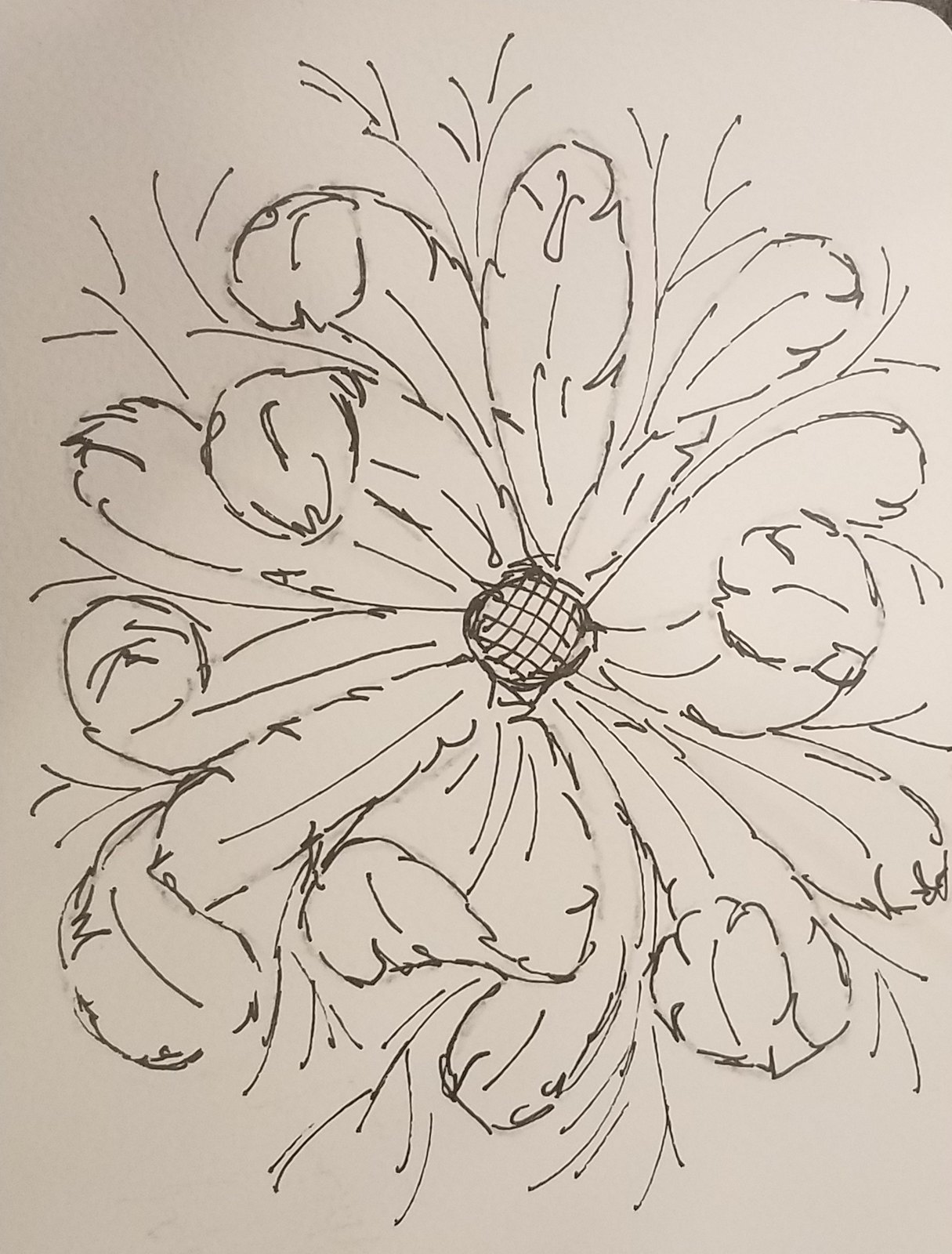This is a photograph of a black and white pen sketch depicting a single, intricately detailed flower. The flower's centerpiece is a circular shape filled with a crisscross or grid-like pattern, suggestive of cross-hatching. From this central circle, roughly ten or more delicate, feather-like petals extend outward. These petals are depicted with light, curly lines, giving them a fluffy and airy appearance as they curl and fold in various directions. The image also features some long, straight leaf-like stems branching out from between the petals, adding to the overall composition. This entire sketch is set against a light gray background, emphasizing the delicate black ink lines that bring this floral design to life.